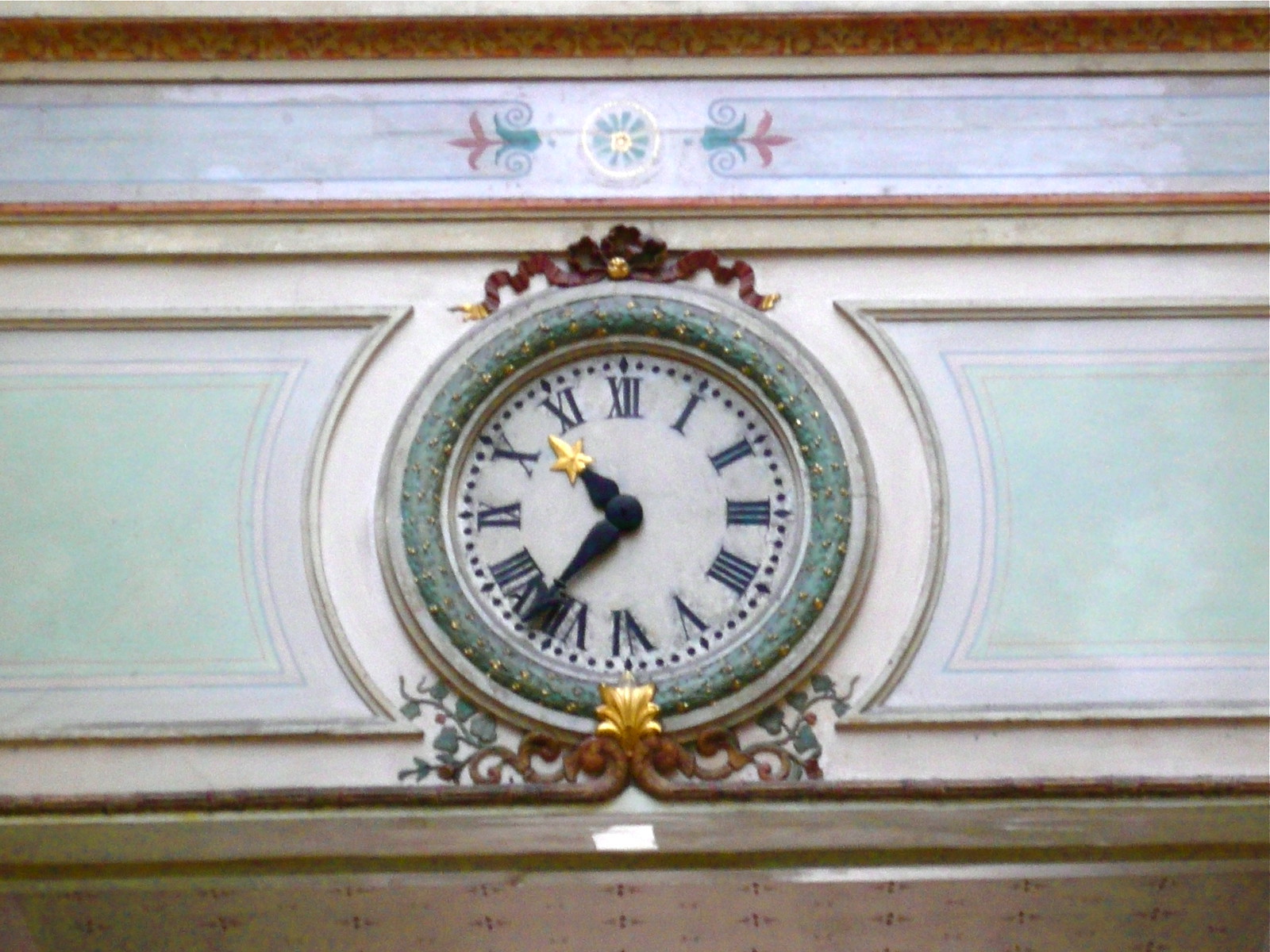A detailed close-up photograph showcases a vintage clock embedded in a wooden structure, possibly part of a dresser or larger piece of furniture. The clock's frame and surroundings exhibit intricate designs at the top, all crafted from wood in a predominant white hue. The clock’s face is a striking teal green, adorned with subtle, sparkling gold accents. The time is displayed using classic Roman numerals, reminiscent of old-school timepieces, with "X" and "I" prominently visible. The black hands of the clock are delicately crafted, and one of the hands, likely the hour hand, is uniquely topped with a small star.